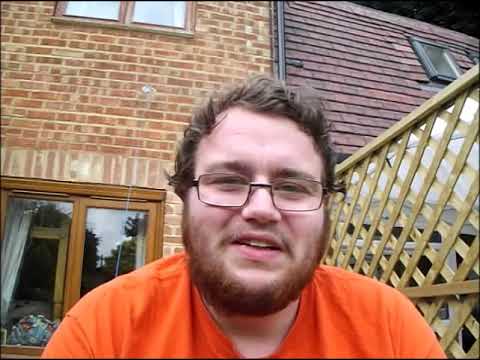In this image, a man in his late 20s or early 30s is captured from the chest up, seemingly engaged in a conversation, possibly on a video call or a vlog. He is a Caucasian male with short, slightly disheveled brown hair, wearing brown-framed glasses, and sporting a medium-length reddish-brown beard and mustache. He is dressed in an orange t-shirt and appears to be either speaking or listening intently, with a slight smile on his face.

The background reveals part of an outdoor setting where he is positioned in his backyard. Behind him, there's a two-story building with sections of brown brick and brownish-red roof tiles, separated by a wood slat fence. The building features a window with a wood border on the first floor and windows with red trim on the second floor. Additionally, next to this structure is another building with a red exterior, black-trimmed windows, and a white umbrella is also visible. The scene suggests a daytime setting, albeit overcast, as indicated by the diffused lighting and reflections in the windows. Numerous items are visible in the windows of the building behind him, adding to the lived-in appearance of the space.